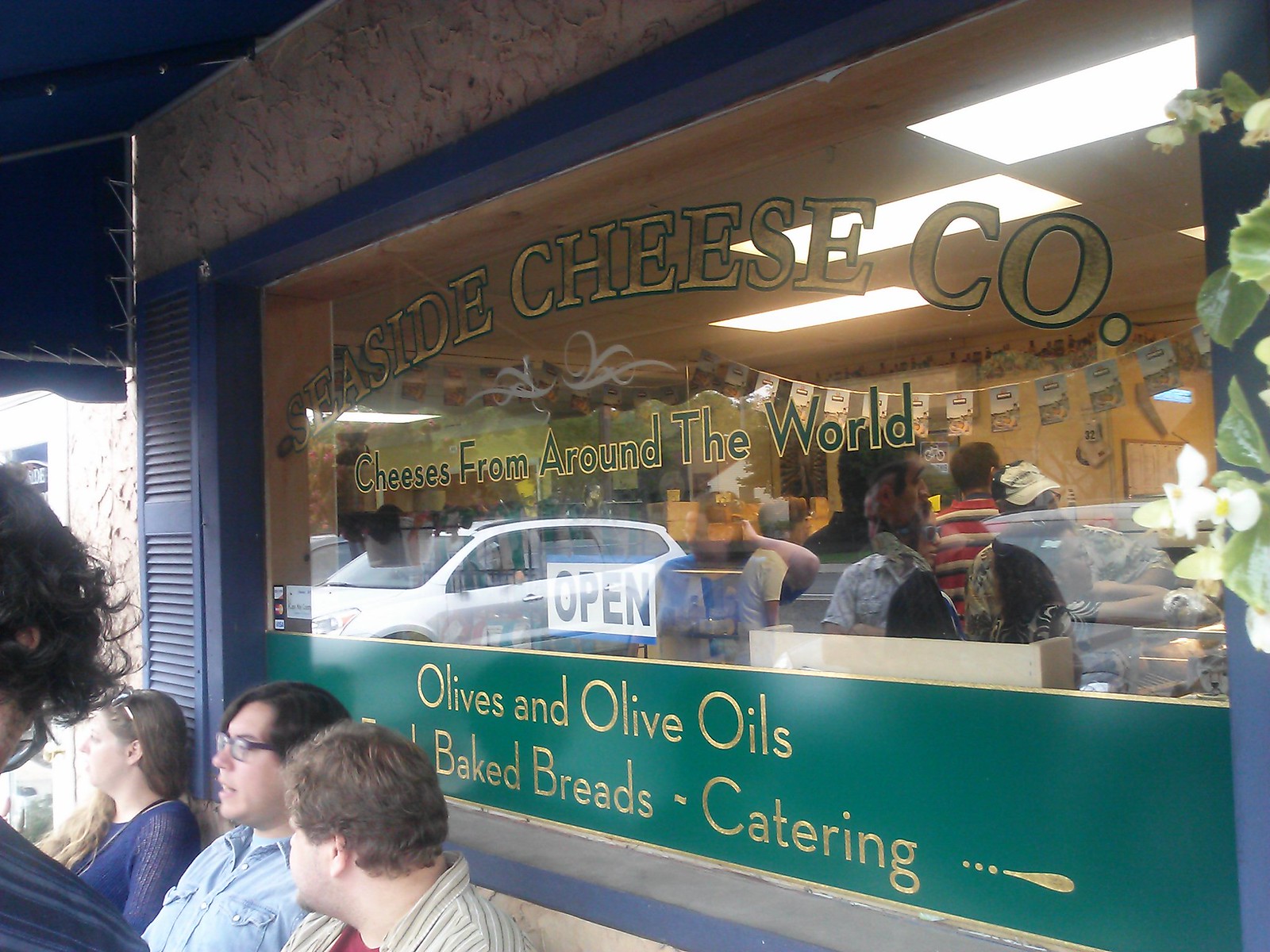The image showcases the storefront of Seaside Cheese Company, highlighting its glass window framed by a blue wood border and blue decorative shutters. The window displays gold lettering that reads "Seaside Cheese Company, Cheeses from Around the World," with additional text below advertising olives and olive oils, baked breads, and catering services. The window features an "Open" sign and reflects a parked car. Inside the store, people are seen ordering items. The building exterior includes a textured stucco or clay wall, a blue awning casting some shadow, and several banners and lights decorating the interior. Outside, three people—a woman and two overweight men—sit against the wall near the window. Additionally, a fourth person, with curly hair and wearing glasses, is partially visible.